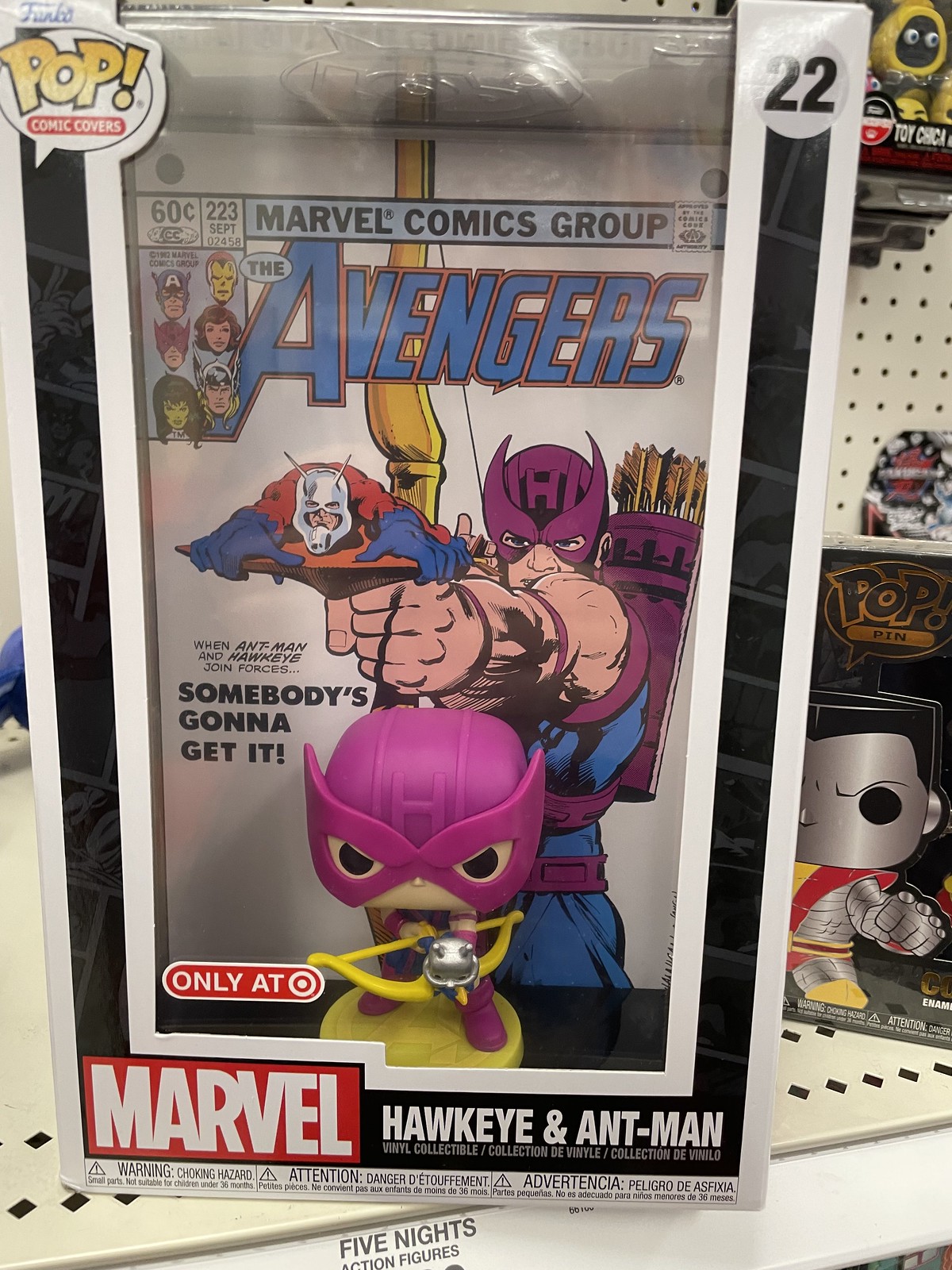The photograph captures a store shelf featuring a boxed Funko Pop toy prominently displayed. The box has a distinct design with a black frame around the clear plastic display window, allowing a full view of the figurine inside. At the top left corner of the box, the word "Pop!" appears in bright yellow font, and next to it, in a speech bubble, "Comics Covers" is written in white against a red background. 

The box features Hawkeye as a plastic figurine, complete with a purple helmet and a purple and blue suit, holding a yellow bow and arrow. Notably, a tiny Ant-Man figure is perched on the arrow. The bottom left corner of the box displays the Marvel logo in white letters on a red background, while the bottom right side features "Hawkeye and Ant-Man" in white letters on a black background, along with a "Only at Target" logo.

Behind the figurine, there is a comic book-themed backing showcasing an iconic Avengers comic cover. The cover features Hawkeye in his classic costume — a purple and blue uniform, gold arrows in a purple quiver, and an active pose as he shoots an arrow. The comic details, such as "Marvel Comics Group," "60¢," "No. 223," and "September," are clearly visible, lending an authentic comic book ambiance to the display.

On the shelf around this main box are other Funko Pop figures, with glimpses of characters including one metallic figure with black eyes, red and yellow accents, and several others positioned on the top right, adding context to the store's broad collection. "Five Nights Action Figures" signage and other descriptive tags are also visible, contributing to the setting as a well-stocked store shelf.